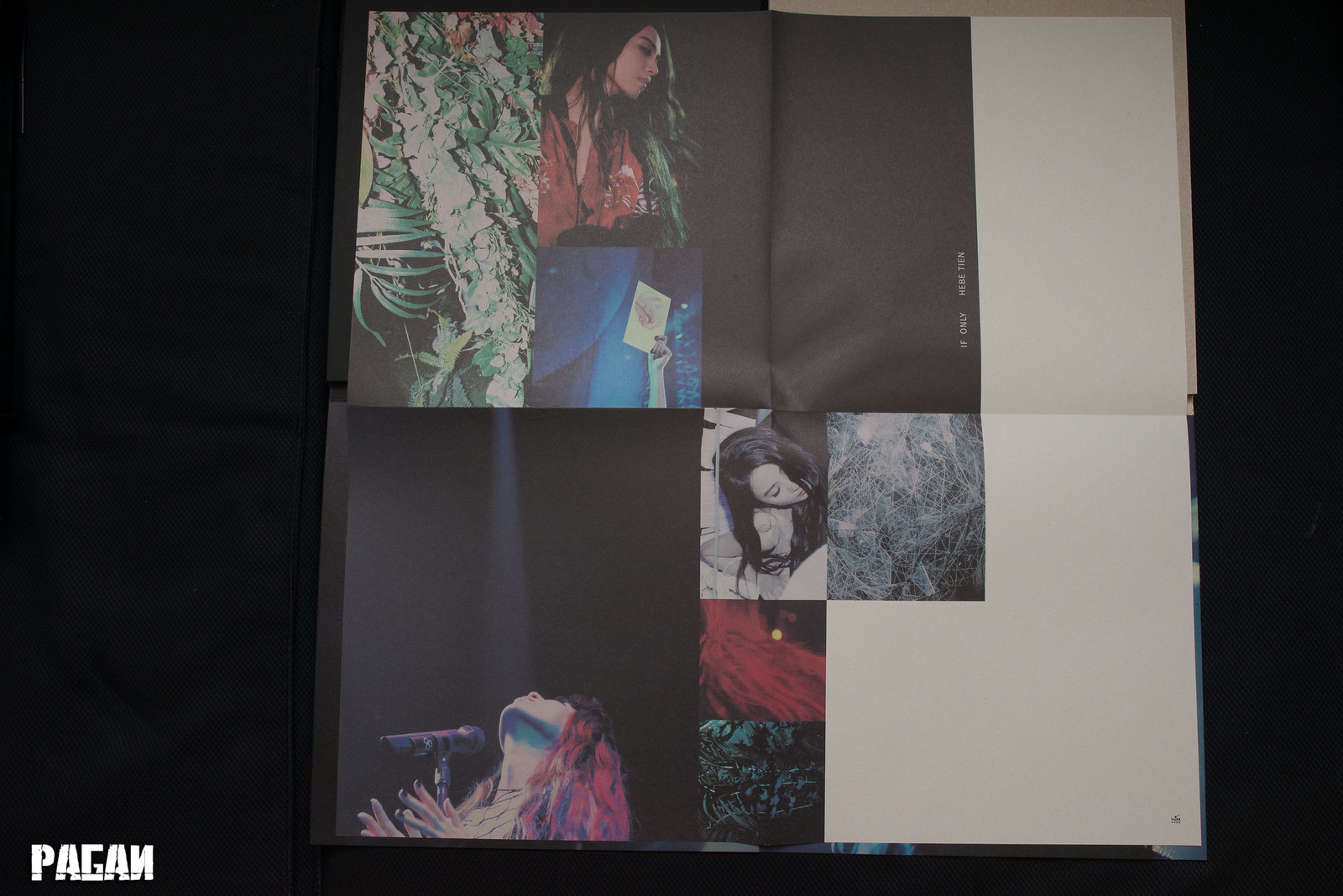The image features an open picture book set against a completely black background. Positioned in the lower left-hand corner is the word "PAGAN," written in white, all capital letters. The book itself appears to have a black binding and is oriented sideways. Within its pages are several photographs, primarily in color but framed by black and white borders. 

On the top left page, there are various depictions within a sort of collage. One picture shows a woman with long black hair wearing a red shirt. She is looking to the right, offering a profile view. To her left is an image of leaves, and below, set against a blue background, a hand is holding up a piece of paper. 

On the opposing page, towards the bottom, there are more photos of the same woman. She is standing in front of a microphone with her head tilted back, her hands gripping the microphone stand. Adjacent to this image are more leaves, and above that is a picture of the woman lying down. Next to this, there appears to be an image of leaves possibly covered in cobwebs. This half of the page continues the pattern of bordered images, some in white and some in black. Across all images, the woman's distinct long black hair and red shirt are a consistent element, with various depictions of her in different poses and settings, including one where she appears to be singing or performing.